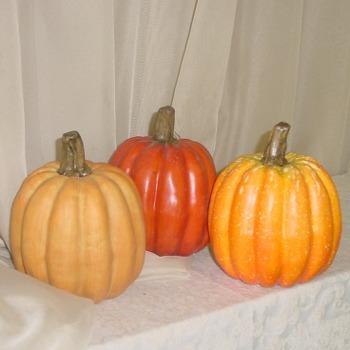The photograph captures three pumpkins with very thick stems and deep grooves along their sides, arranged on a white slab. The slab appears to be draped with a white cloth, potentially lace with another light-colored fabric underneath. Each pumpkin exhibits a unique shade: the left pumpkin is a pale, slightly orange hue; the center pumpkin is a rich, shiny, red-orange; and the right pumpkin is orange with a hint of green near its slightly bumpy stem. These pumpkins, which might be artificial due to their glossy, almost plastic appearance, stand before a white, slightly translucent curtain that could be composed of two pieces of fabric pulled together. The overall scene has an air of meticulous arrangement, casting doubt over the pumpkins' authenticity due to their shininess and painted-looking stems.